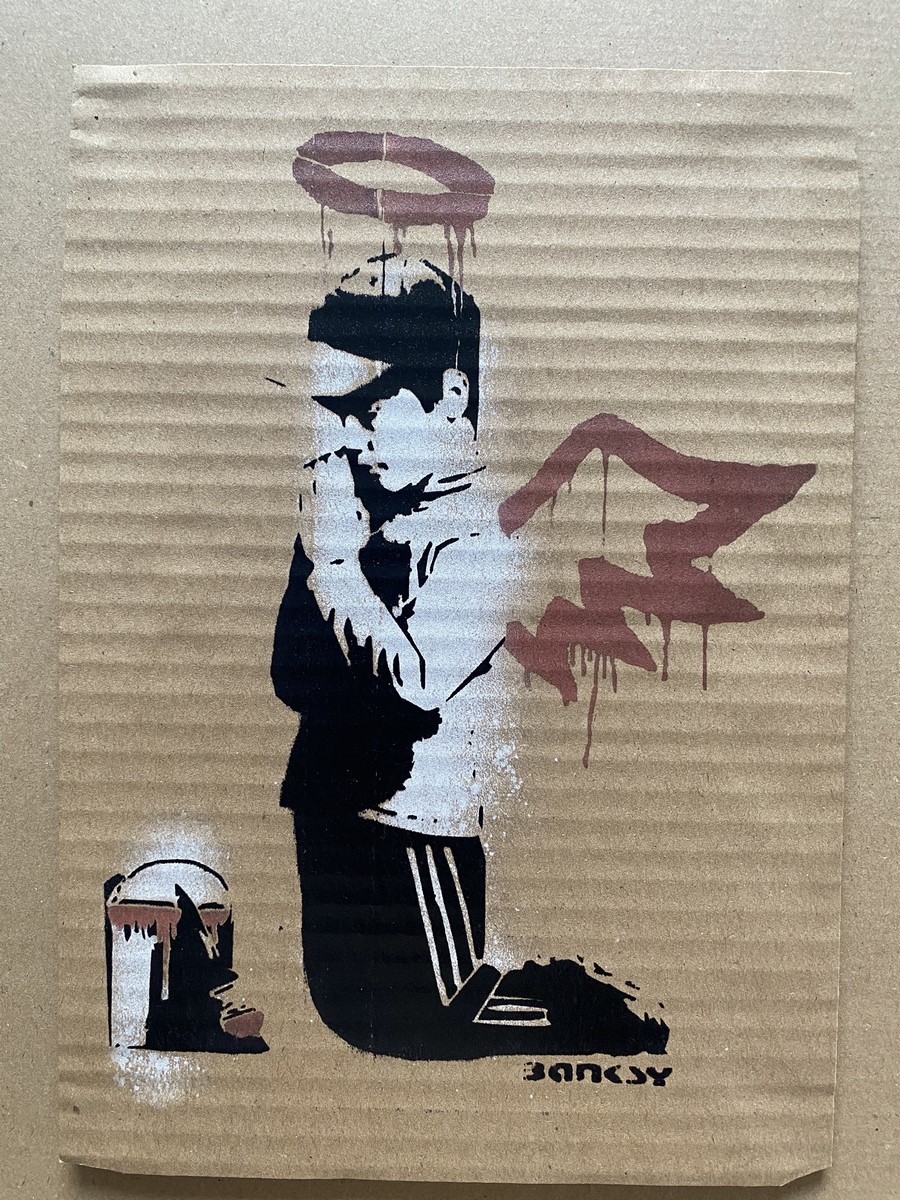The image depicts a detailed sketch on a square piece of light brown cardboard, possibly folded, serving as a textured background. The focal point is a young person, likely a boy, characterized by black hair and striped black and white pants, kneeling in front of what appears to be a pew with a cushioned kneeler. He is depicted in a praying position, with his hands together in front of his face and a halo hovering above his head, suggesting sanctity. A brown wing is drawn behind him, enhancing the angelic imagery. The boy wears a black hat, and a paint bucket with a paintbrush is placed on the ground nearby. The contrast of black and white within the drawing, especially notable on his hands and shirt, adds depth and emphasis. Notably, the name "Banksy" is inscribed beneath the kneeling figure, identifying the piece as the work of the renowned street artist, Banksy. The natural lighting in the scene ensures that all elements are clearly visible.